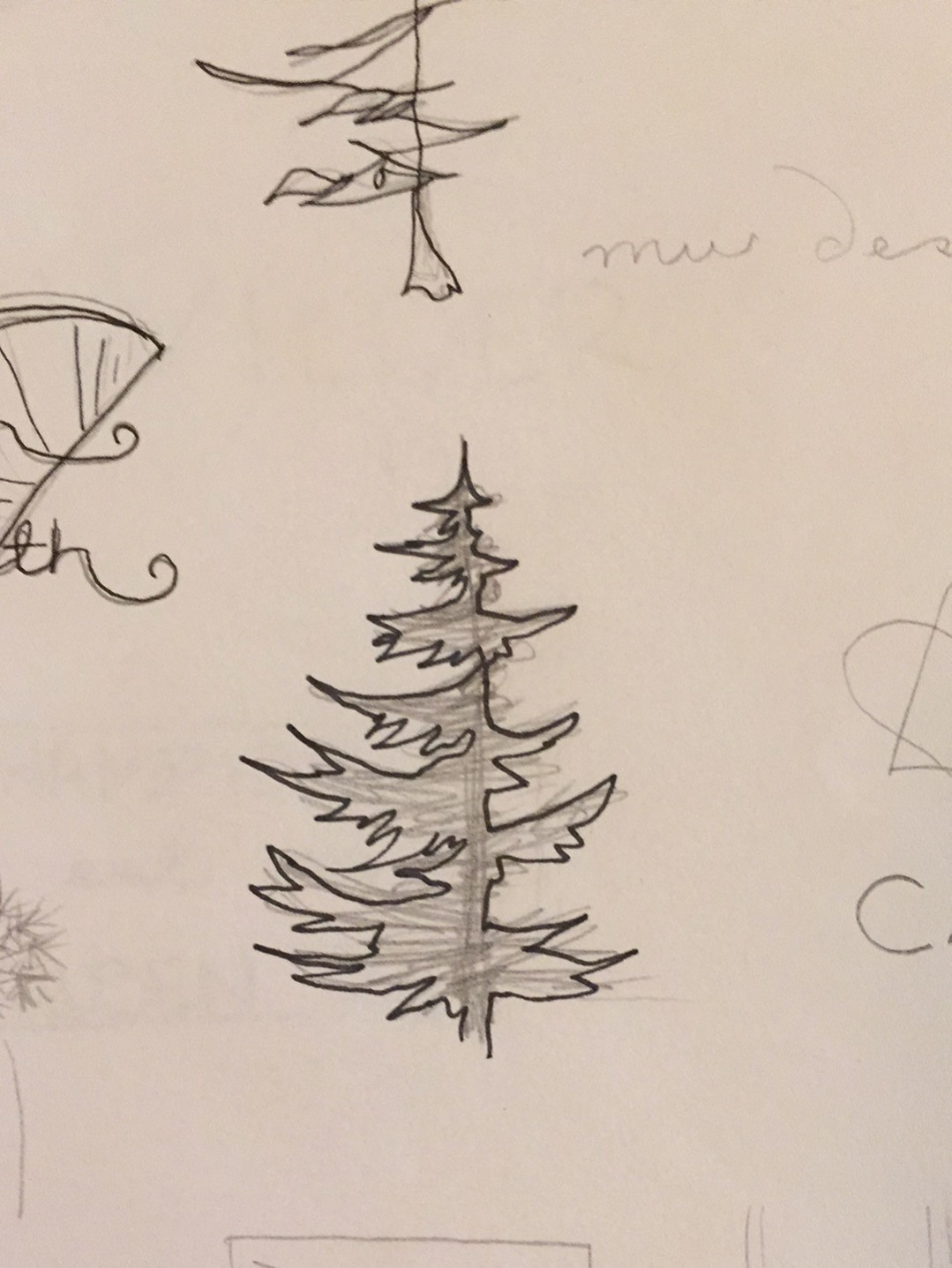This photo captures a close-up of a white piece of sketch paper scattered with various drawings and writings in both black pen and grey pencil. At the center of the paper stands a prominent fir tree, outlined in black pen with a rough, scribbled shading of grey pencil inside, giving it a hurried and messy appearance. Above the tree, there are squirrely lines that resemble a mast with a pennant or perhaps an obscure plant-like design. To the right of the tree, a large 'C' is visible, alongside cursive writing that begins with "M-U" followed by "D-E-S," possibly spelling out 'murder.' On the left side, partially cut off, is a wedge-shaped object with the letters "TH" in cursive at its base. The bottom center features half of a rectangle, further adding to the chaotic assortment of lines surrounding the tree, most of which appear to be random and without recognizable form.